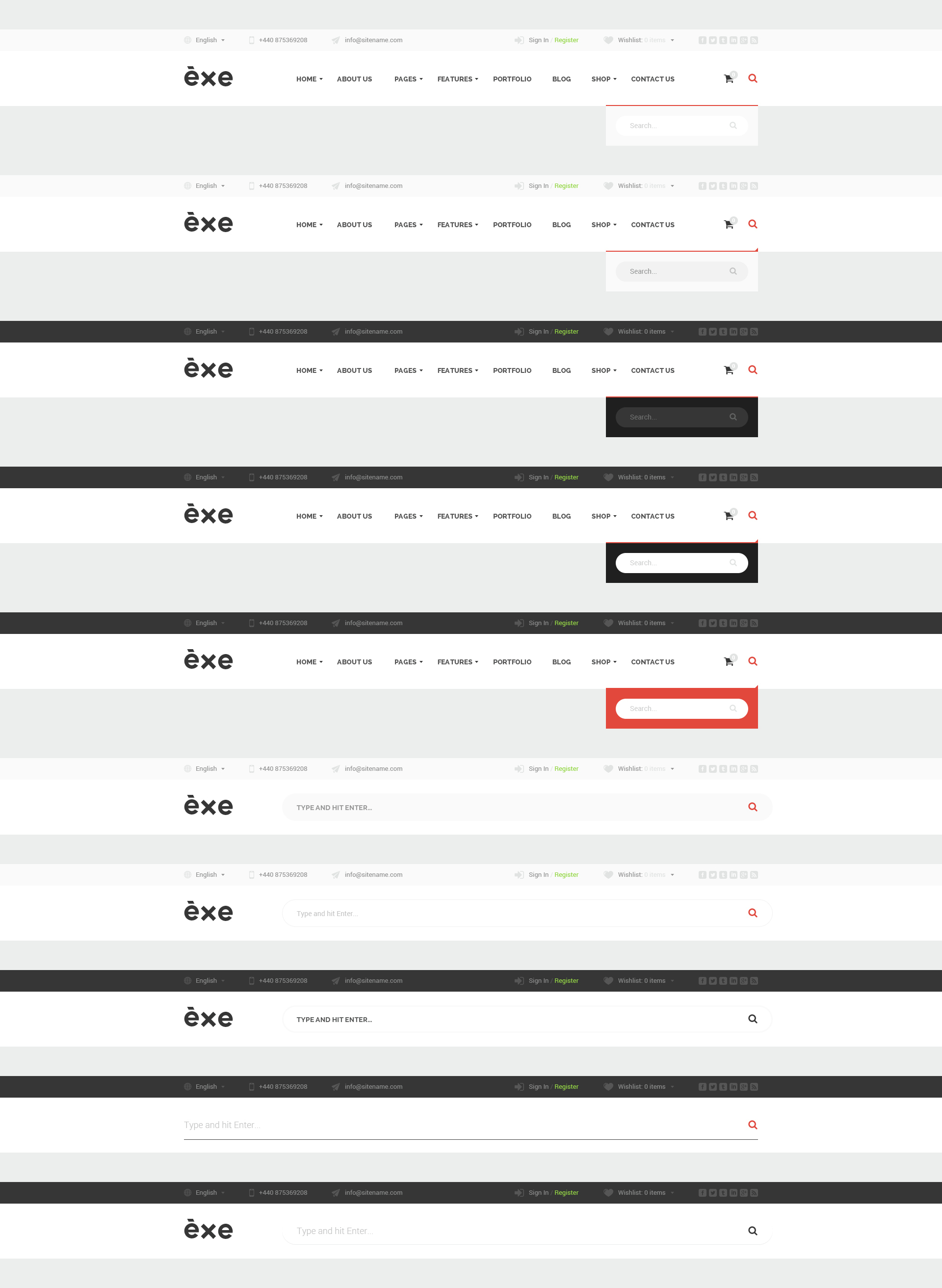The image showcases a cluttered web page view, featuring multiple overlapping instances of the same website, identified as "exe." The primary web page displays a navigation bar equipped with various options including language selection (English), a phone number, the website URL, sign-in and register buttons, a watch list, and other home navigation options such as Home, About Us, Pages, Features, Blog, Shop, and Contact Us. Additionally, it includes a shopping cart icon and a small search button located at the bottom right corner, which appears in different color variations – black and white in one instance, and red and white in another. The image depicts 9 to 10 overlapping instances of the "exe" website, creating a complex and somewhat chaotic visual of repeated web page layers, providing no substantial information to clarify its intended purpose or function.